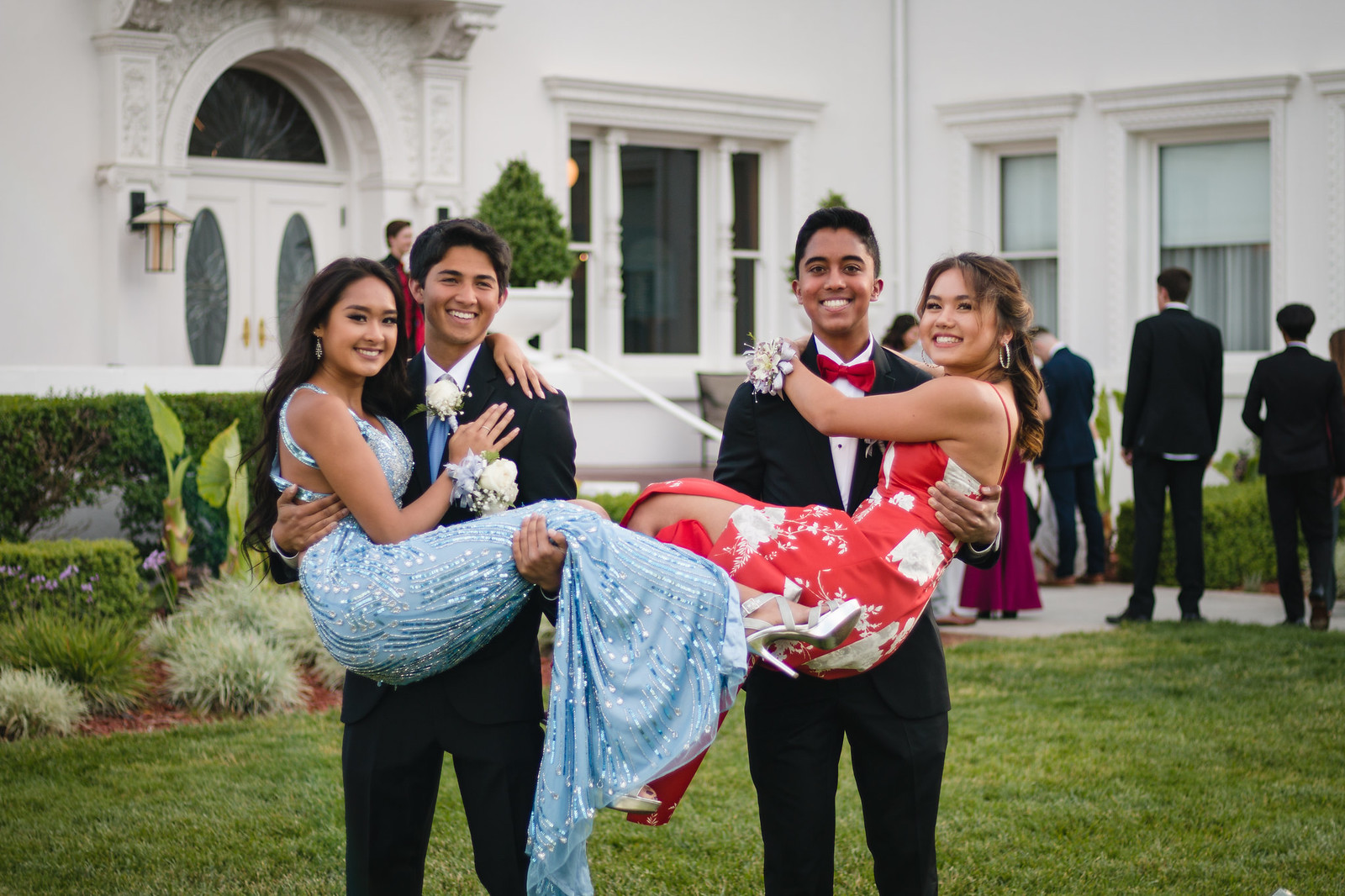This photograph captures a joyful moment before prom night, showcasing two young couples posing in front of an elegant home. The two young men, dressed in black suits, are each holding a young woman in their arms. One man sports a blue tie, while the other complements his attire with a red bow tie. Both women are adorned in long dresses; one wears a striking blue sequin dress paired with open-toed high heels, and she has long black hair. The other woman, with long dark brown hair, dons a Hawaiian-style red and white dress. The backdrop features the elegant facade of a house with visible windows and is accented by green grass and plants. The scene suggests a festive occasion, likely a prom or high school dance, given the formal attire and corsages on both young women. Additionally, other teenagers in suits can be seen in the background, enhancing the celebratory atmosphere. The image reflects a blend of excitement and elegance, typical of a significant social event for these teenagers.